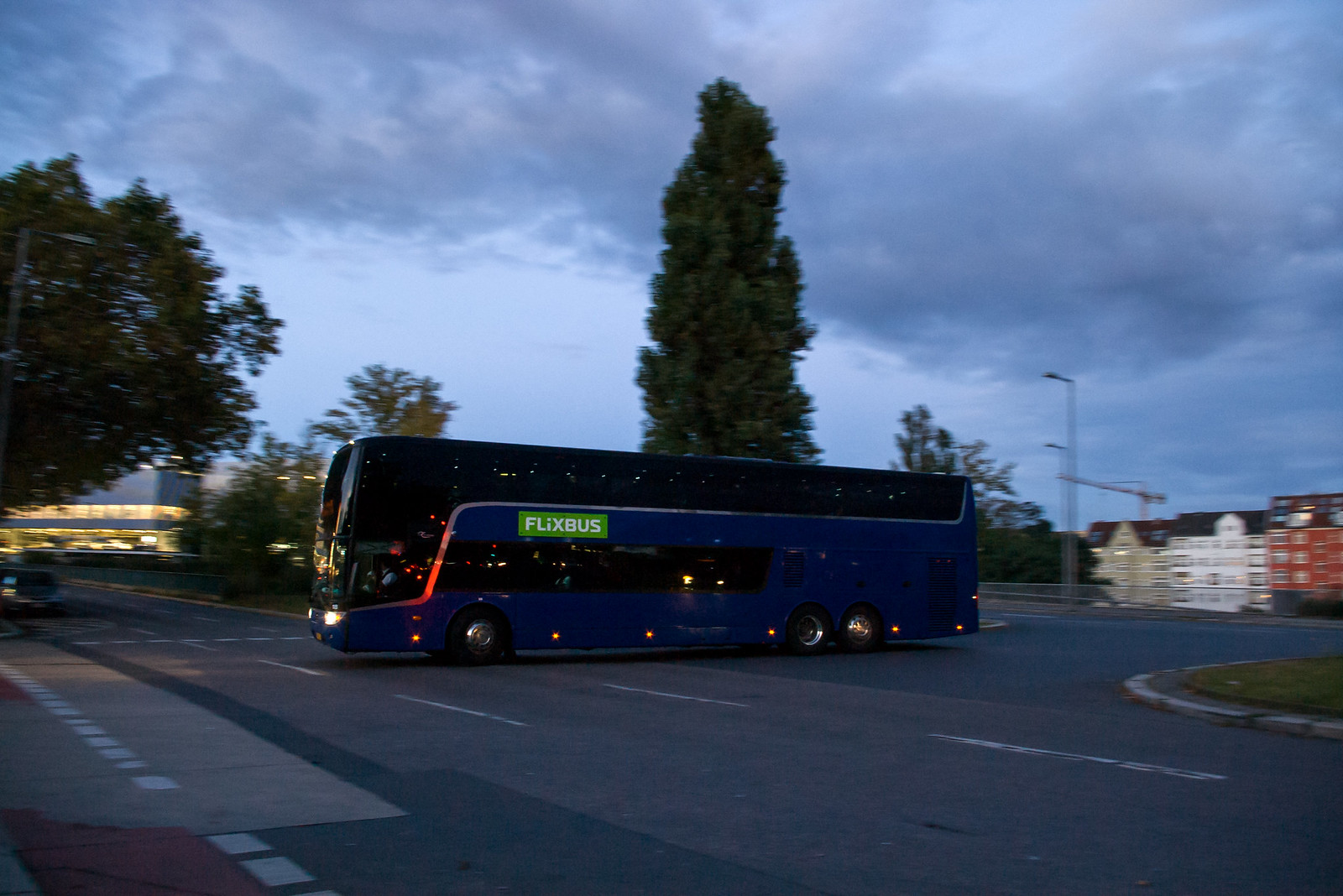This image captures a sleek, double-decker bus, painted a dark blue with black-tinted windows. Prominently displayed along the side of the bus is a green banner emblazoned with white letters spelling out "Flixbus." The bus, captured in profile, is depicted parked across multiple spaces in a parking lot, with the empty gray street suggesting a quiet evening or dusk setting. The scene is set against a backdrop of towering trees, including a notably large spruce, with hints of urban infrastructure such as street lamps and distant residential buildings and an office building illuminated from within. The sky overhead is a darkish blue, further suggesting the approach of night.